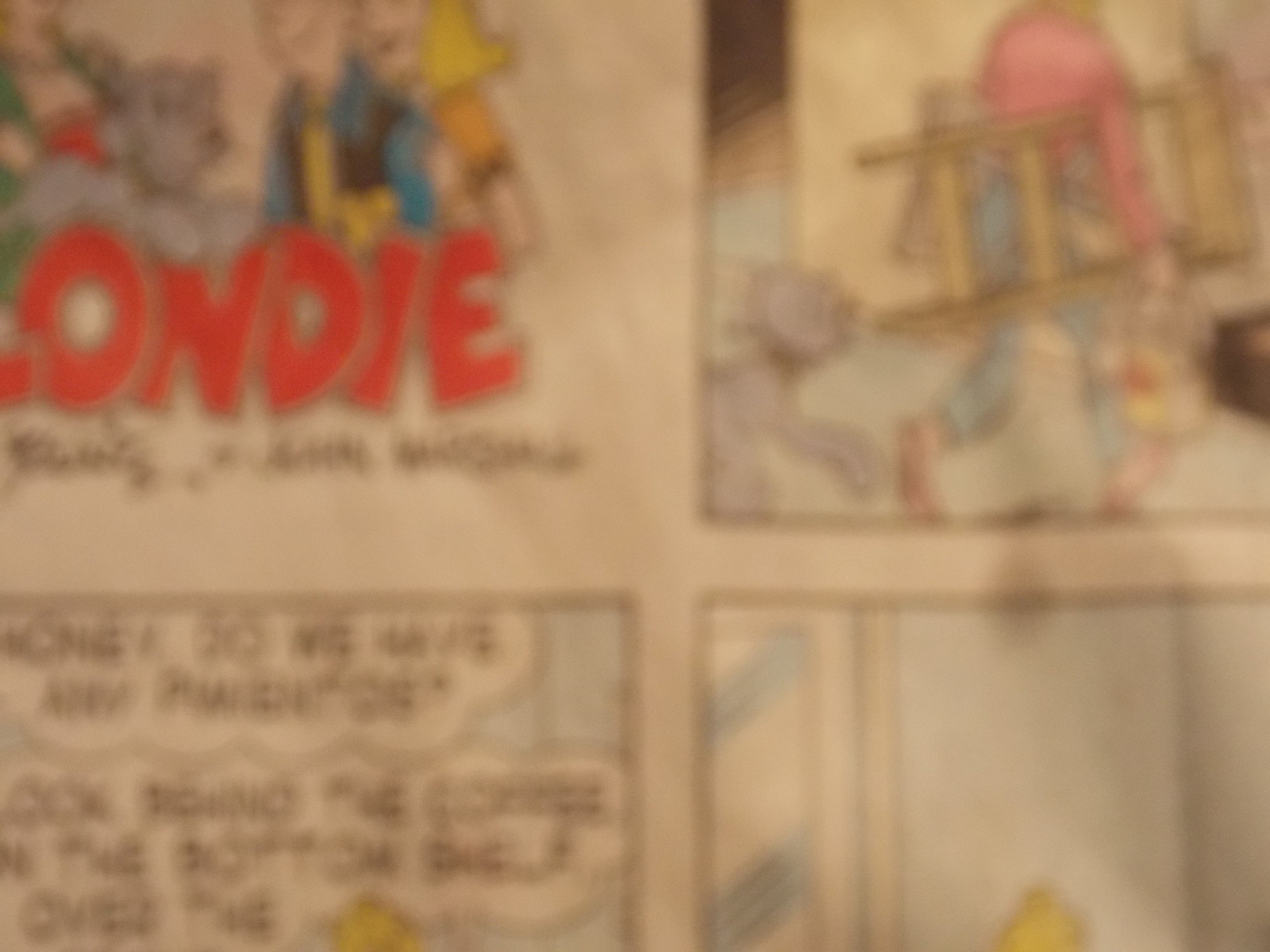This blurry close-up view captures four partial panels of the comic strip "Blondie," rendering its content barely recognizable. In the top left corner, a fragment of the bold red title "Blondie" is visible, alongside partial images of a dog, a woman, and a man. The top right section shows a person carrying a ladder and a can of paint, with a dog trailing behind. The bottom left portion features several indistinct conversation bubbles, their text obscured by the blurriness. Finally, the bottom right displays a fragment of a wall and door. The image's lack of clarity makes it challenging to discern finer details or follow the narrative.